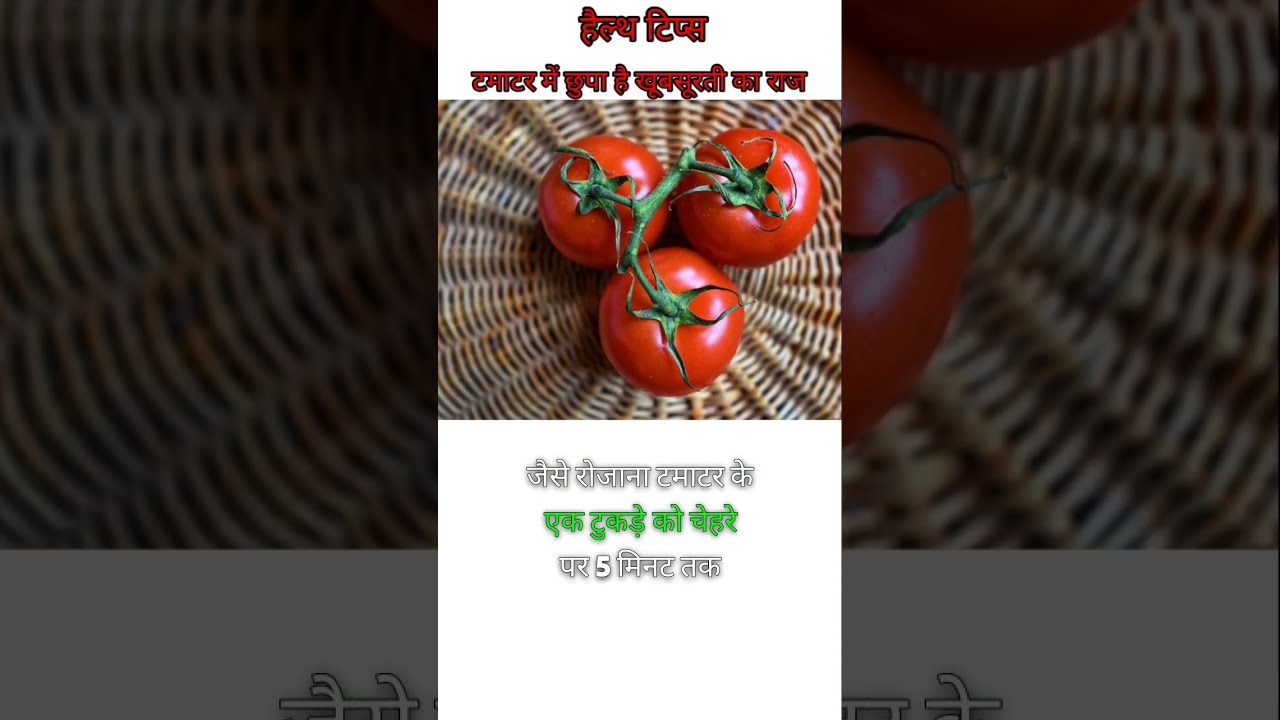The image features a top-down composition of three vibrant red tomatoes still attached to their bright green vine, arranged in a triangular shape. These tomatoes rest on a circular, woven wicker basket that exudes a rustic, farmer's market feel. The background of the image consists of the brown woven material of the basket, providing a contrasting backdrop to the vivid red tomatoes.

Above the main image, written in a red font with a black outline and set against a white background, is text that appears to be in Arabic. Below the tomatoes, also on a white background, are three lines of text, where the first and third lines are in white font, and the middle line is in green, with some text recognizable as the number five.

The left and right sides of the image are adorned with magnified and tinted close-up shots. The right side shows an enlarged portion of a tomato, while the left side features a close-up of the wicker basket. These superimposed sections frame the central composition, adding depth and focus to the primary subjects in this portrait screengrab orientation.